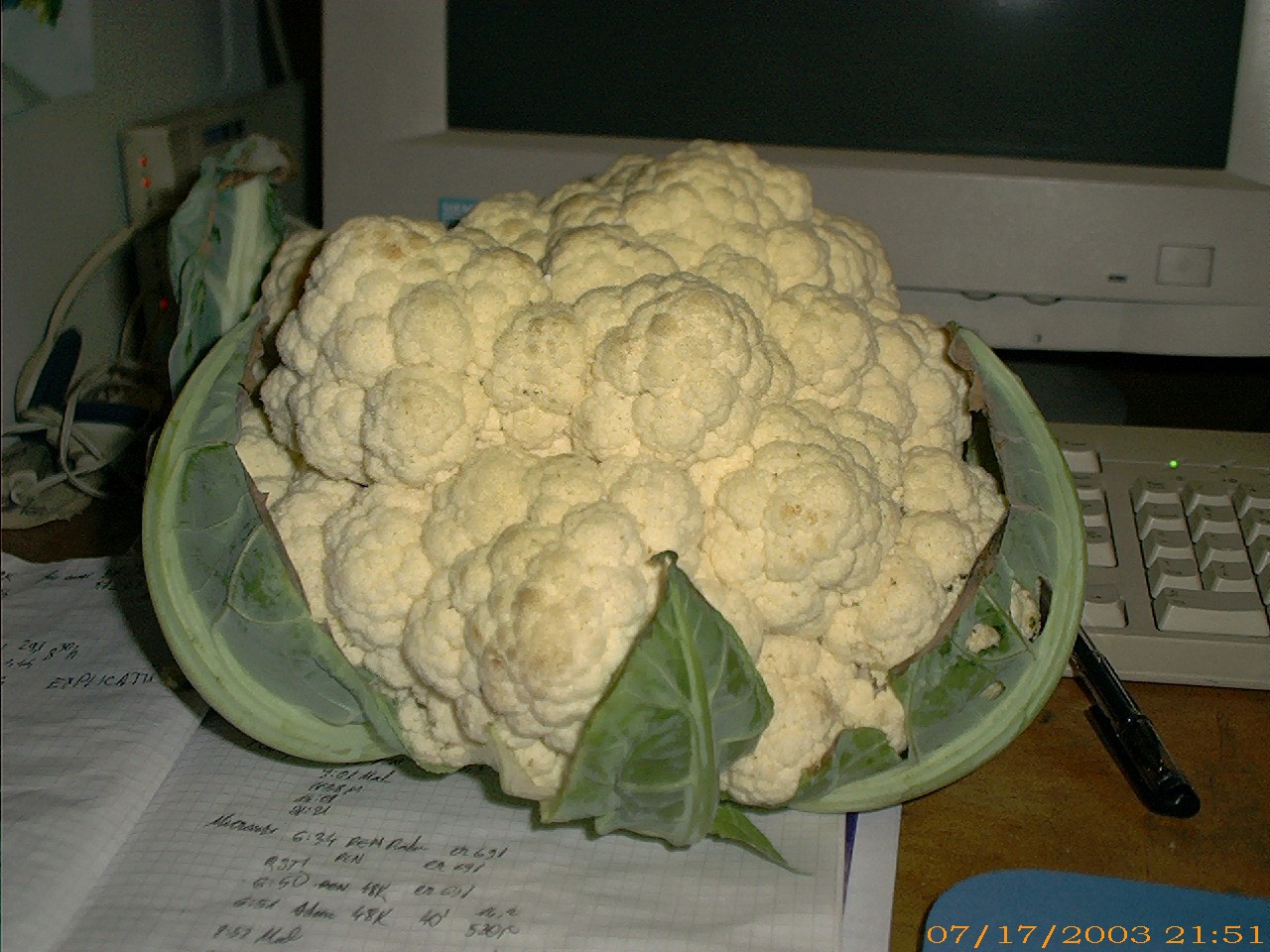This color photograph features a close-up view of a head of cauliflower placed prominently at the center. The cauliflower is light yellow with several darker beige spots scattered on its top and front face, indicating it's a few days old and should be cooked soon. The texture is clustery and fluffy, composed of small lumps that form medium-sized clusters. Surrounding the cauliflower, three dark green leaves curl up around the head. These leaves are slightly ruffled with pointed ends, intricate veins, and lighter green striations.

The cauliflower rests on an open notebook filled with grid paper, displaying various handwritten text in black ink, suggesting math problems or notes. Behind the notebook, a vintage computer setup is visible. The bottom half of an old-school computer monitor with a white plastic frame and black screen stands right behind the cauliflower. Below the monitor, a matching white plastic keyboard is visible. In the backdrop, part of a medium-brown wood grain desk or tabletop can be seen, along with the capped side of a black pen.

The image is also timestamped in the bottom right corner with yellow text reading "07-17-2003; 21:51," hinting at the date and time the photograph was taken, thereby placing the scene in an early 2000s timeframe.